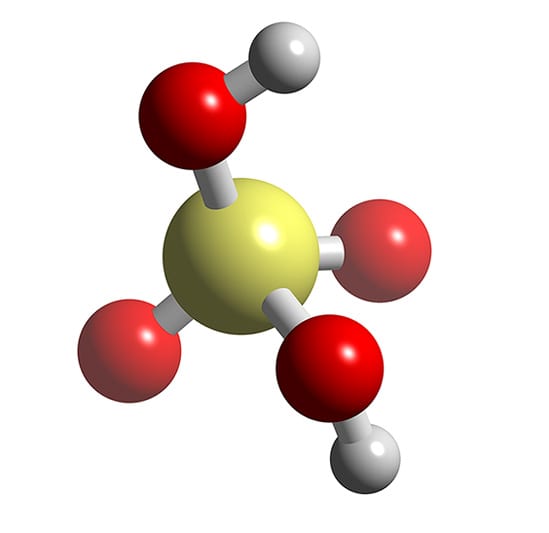The image is a detailed computer-generated illustration of a molecule, reminiscent of a chemistry set model. At the center is a large, shiny yellow ball with a slight white glare, symbolizing possibly a nucleus or central atom. Protruding from the yellow ball are four white cylindrical connectors attaching to four shiny red balls. Two of these red balls have smaller white cylinders extending from them, each leading to a shiny, smaller gray ball. The gray balls are positioned such that they create an intricate structure, giving an impression similar to an atomic or molecular model with a striking resemblance to those used in educational settings to demonstrate molecular compositions.